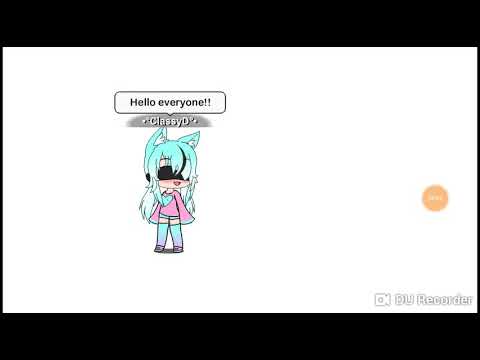The image is a rectangular screenshot from a cartoon featuring a chibi anime-style character positioned in the center left, standing against an all-white background. There are black bars at the top and bottom, giving it a letterboxed appearance. In the bottom right corner, there is a logo that says "DU Recorder" alongside a small yellow circle with unreadable text, and an icon that resembles a video camera.

The character, a young girl, is drawn in an anime style reminiscent of a caricature, with cat ears, long teal hair that reaches her waist, and a black blindfold around her eyes and nose. Her mouth peeks out just below the blindfold. She is depicted wearing a pink top with bell sleeves, teal shorts, and ombre stockings that transition from teal to purple. Her legs are slightly apart, and she seems to be interacting with the viewer. Above her head is a speech bubble that says "Hello everyone!!" with a smaller grey cloud below it that reads "Classy D".